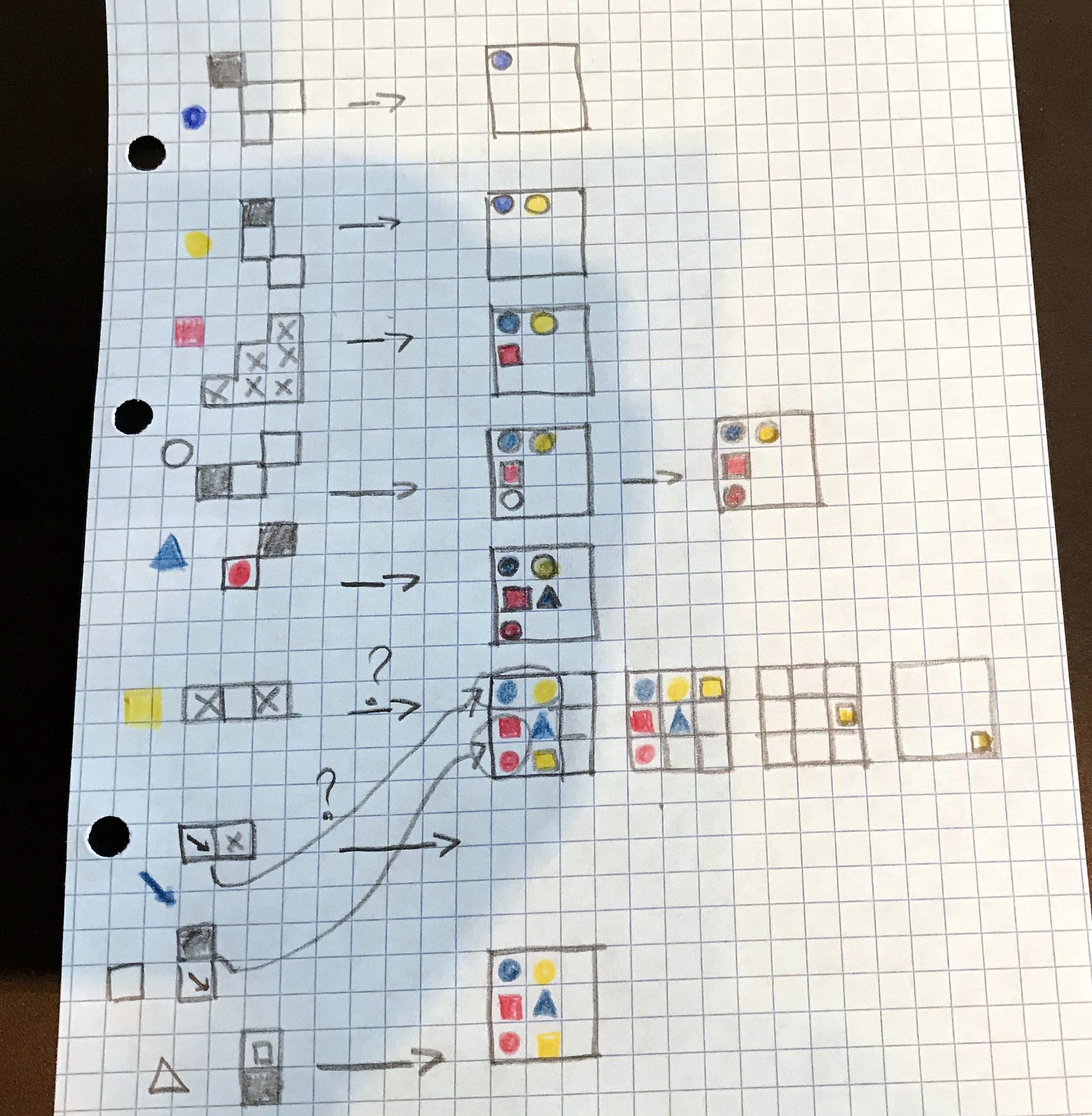This photograph showcases a piece of white graph paper featuring both dark gray and light blue lines, indicating its suitability for detailed drawings or mathematics. The left side of the graph paper has three punched holes, suggesting that it was either removed from or intended for insertion into a notebook. The backdrop for the graph paper is a stark black, providing a clear contrast to highlight its content.

At the center of the graph paper, a series of meticulously drawn squares extends from the top center to the bottom center. Notably, the fourth line from the top includes an additional square off to the right, connected to the central square by an arrow. Two rows beneath this, three more squares extend to the right of the central alignment, each containing various shapes filled with primary colors: blue, yellow, and red.

Along the leftmost side of the graph paper, there is a column of gray-colored shapes resembling Tetris cubes, drawn with a gray pencil. Adjacent to this column, a color key indicates the specific hues corresponding to each shape. Each gray square in this column is connected by a gray arrow to a square within the central lineup, illustrating a clear relationship between the columns. This image captures a meticulous and colorful arrangement, combining elements of structure, connectivity, and artistic expression.